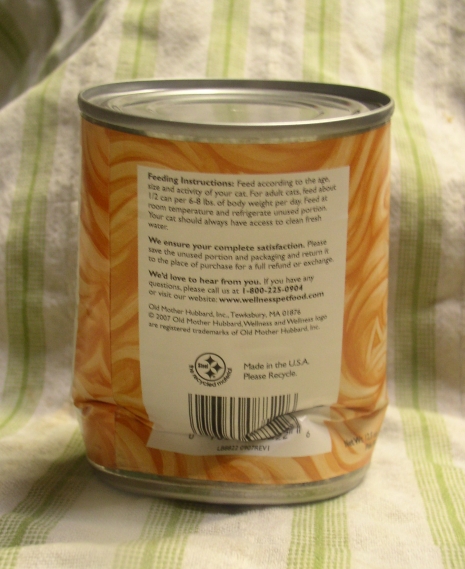A photograph showcases a dented can of cat food placed on a white and green striped towel. The green stripes are noticeably thinner than the white ones, adding a subtle yet distinct contrast to the towel's design. The can itself features a silver-colored top and bottom, and its label displays an orange and white striping pattern. On the back of the label, detailed feeding instructions are printed on a white section, advising owners to feed their cats according to age, size, and activity level. Specifically, for adult cats, the recommendation is to provide about half a can per six to eight pounds of body weight daily, ensuring the food is served at room temperature and any unused portion is refrigerated. Additionally, it emphasizes the importance of giving cats access to clean, fresh water at all times. For complete satisfaction, it advises saving the unused portion and packaging and returning it to the place of purchase for a refund or exchange. For any questions, customers are encouraged to call 1-800-225-0904 or visit wellnesspetfood.com.